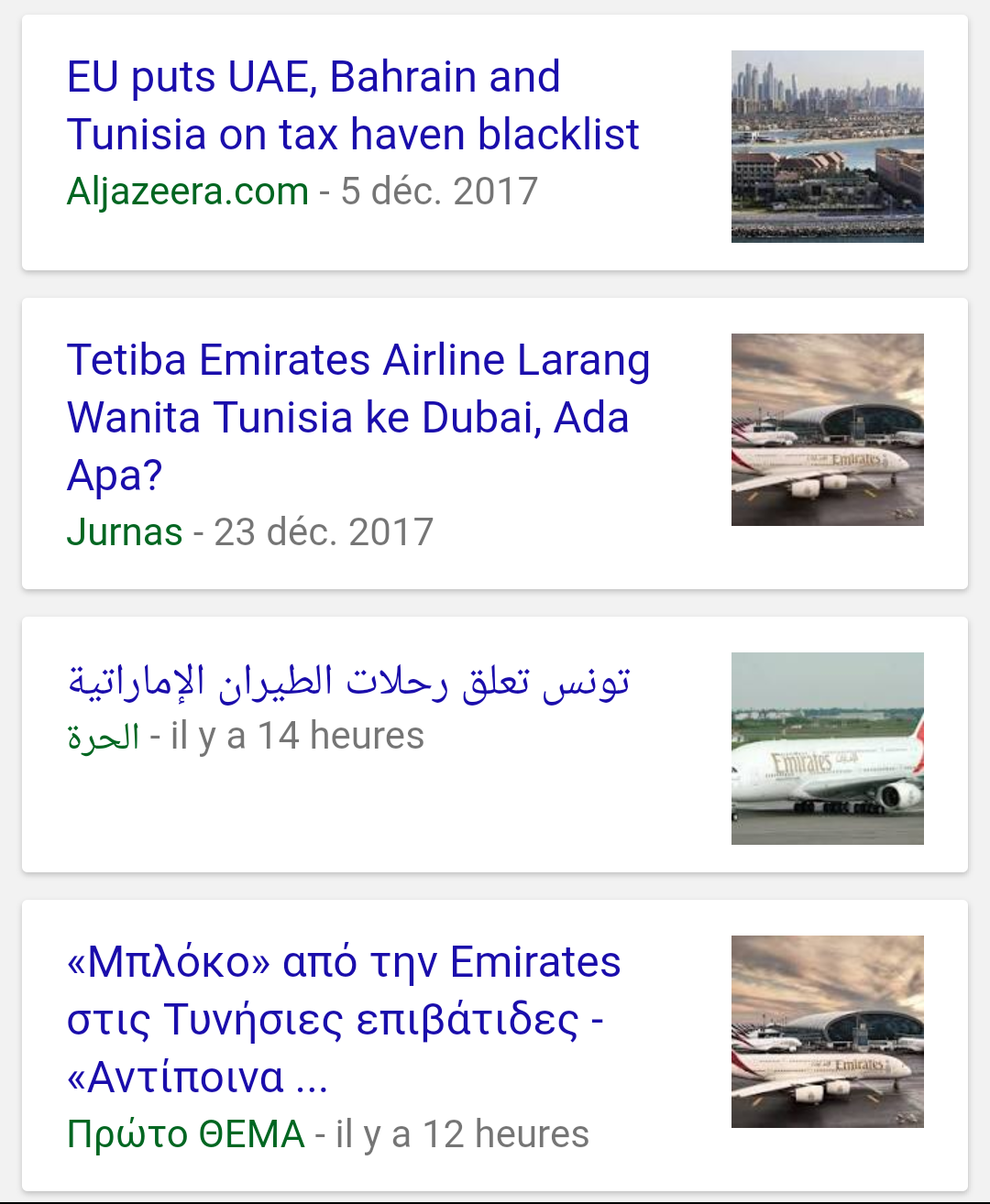This image appears to be a collage of screenshots from various news articles displayed on a Google search tab. At the top, there's a headline reading "EU puts UAE, Bahrain, and Tunisia on tax haven blacklist," with the article sourced from Al Jazeera, posted on December 5th, 2017. Accompanying this article, there's a small image depicting a cityscape. Below that, another headline mentions "Tediba, Emirates, Airline, Laring Wanita, Tunisia, KE, Dubai, ADA, APA." This one is attributed to a site called Jurnas, dated December 23rd, 2017, and is paired with a photo of an airplane. Further down, an article in Arabic features a different plane image. Finally, the bottom entry is in another language but uses the same airplane photo as the second article.